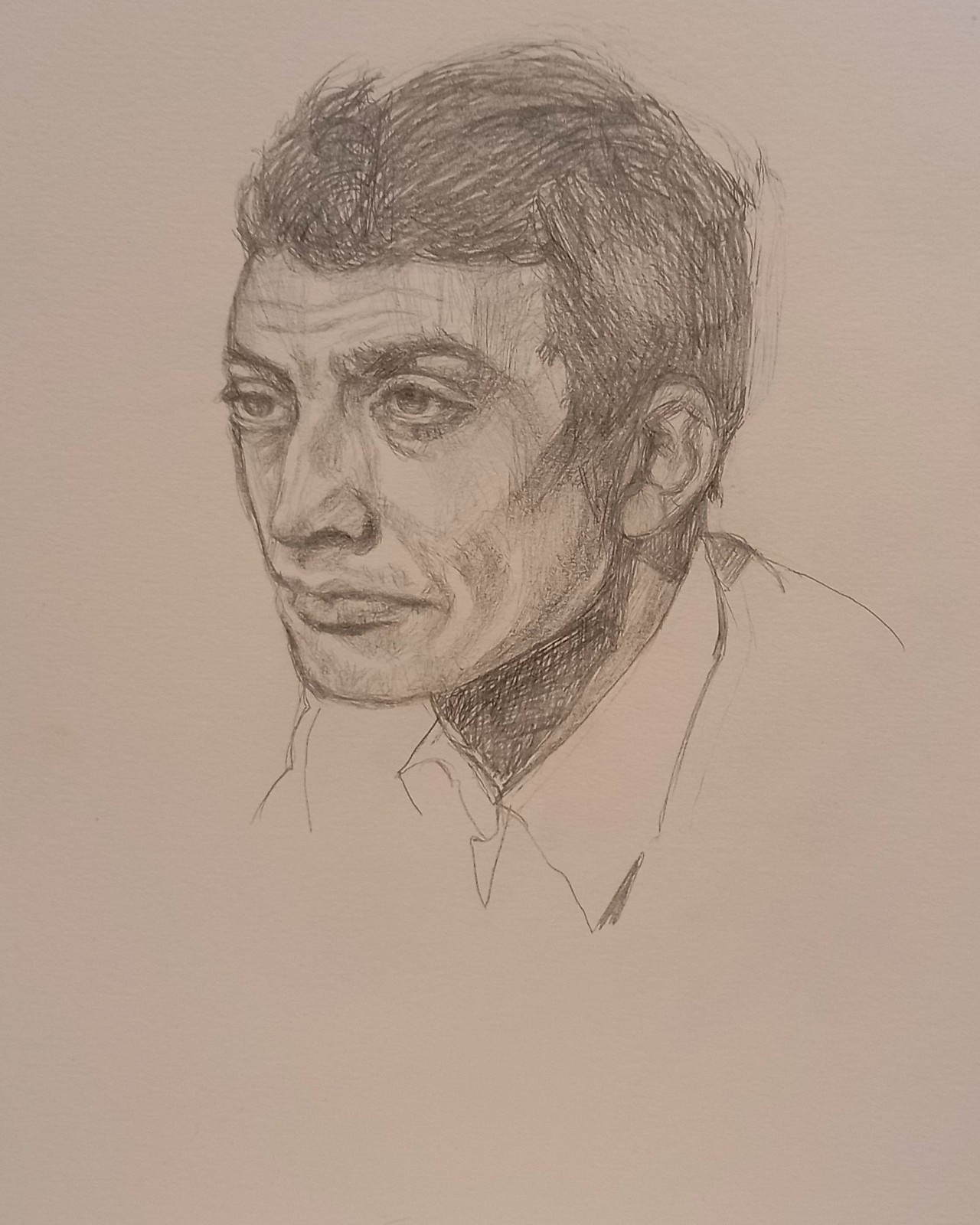A meticulously detailed pencil drawing captures the image of a serious, pensive man. His expressive face shows a wealth of emotion, with bushy eyebrows and a forehead marked by wrinkles. His hairstyle is carefully rendered, appearing gelled at the front, and long enough to reveal distinct sideburns. Notably, his right eye appears slightly smaller than his left, adding a touch of asymmetry to his otherwise symmetrical face. He has a straight nose and very full lips. Underneath his chin, there is extensive shading that creates the illusion of a scarf or heavy shadow, contrasting with the lighter shading on his face. The man is dressed in a collared garment visible in the drawing before it ends. The artwork is crafted on a unique pinkish-gray paper, enhancing its depth and texture.